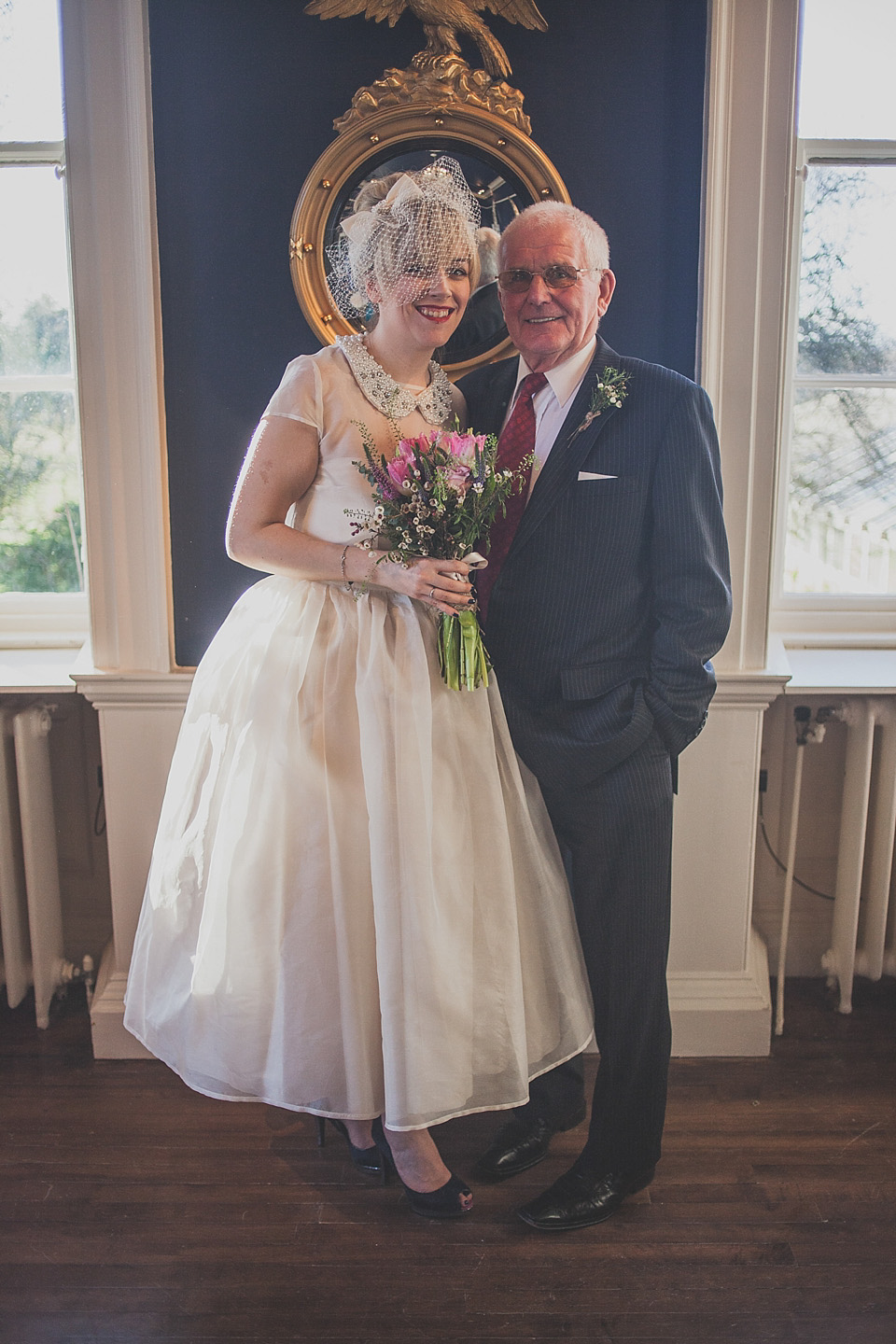In this indoor wedding photo, a bride and an older man, likely her father, are posing together in front of a navy blue wall adorned with a golden-outlined, round decorative piece, possibly a mirror, embellished with what appears to be an eagle at the top. White-paneled windows flanked by white pillars frame the backdrop, and the dark brown hardwood floor adds a touch of elegance to the setting. The bride, a Caucasian woman with red lipstick, is dressed in a short-sleeved, ankle-length white wedding gown, accompanied by a veil that covers her face to her nose. She holds a bouquet of pink and white flowers and wears dark shoes. Beside her stands an older, balding man with white hair and glasses, sporting a dark suit jacket, white collared shirt, red tie, and black shoes. The duo stands close, smiling, with their hands affectionately placed on each other’s backs.